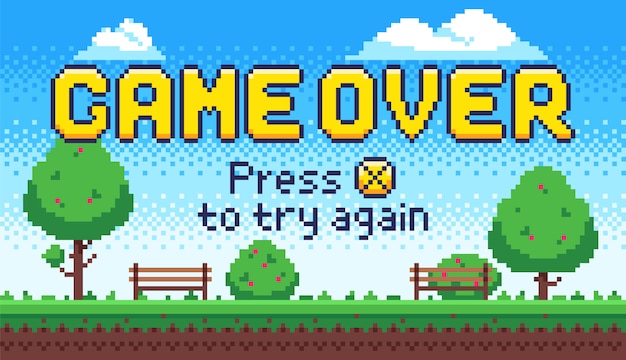The image is a pixelated screenshot from an old-school video game reminiscent of classics like Mario or Yoshi. Dominating the top of the image, bold yellow text outlined in black announces "Game Over." Below it, in smaller black letters, an instruction reads "Press X to Try Again," accompanied by a yellow circle with the 'X' symbol. The scene depicts a park with vivid pixelation: a deep blue sky dotted with fluffy white clouds, green trees bearing red berry-like dots, and a ground layered with green grass over brown dirt. Two brown park benches are spaced out, one on the left and the other on the right, contributing to the tranquil park setting. Despite the detailed environment, no game characters or specific logos are present to pinpoint the exact game.